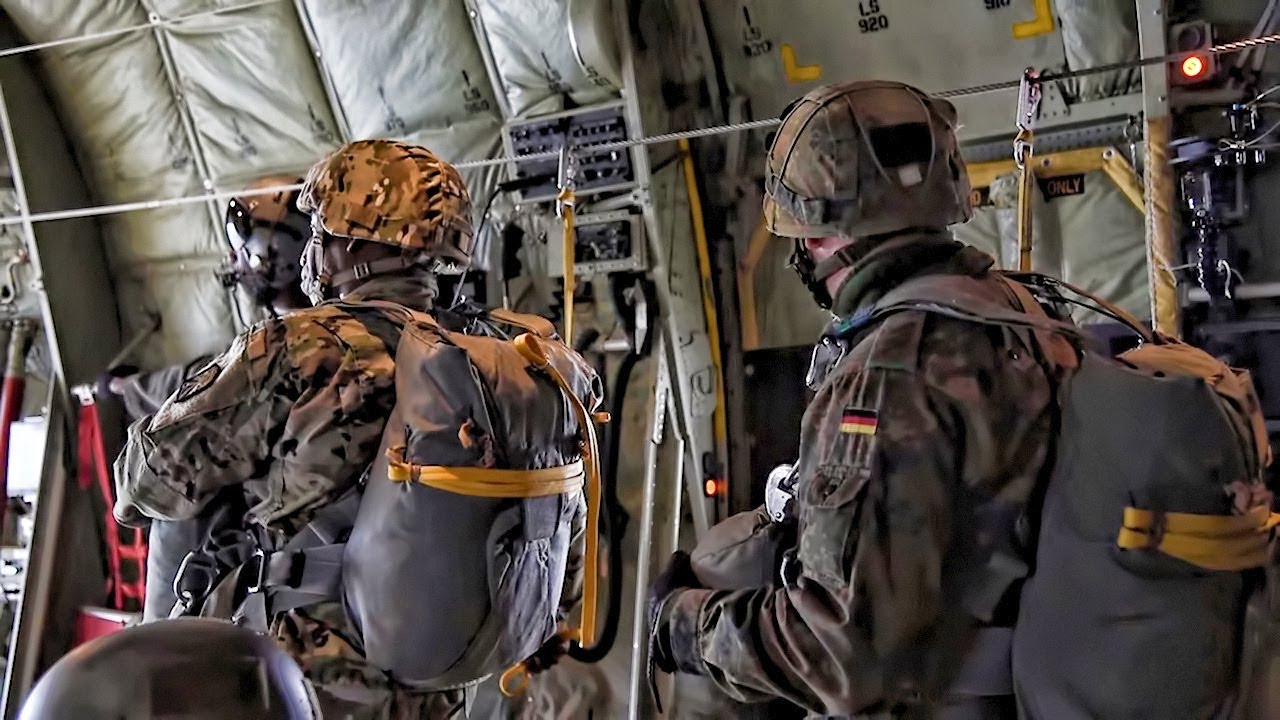In this color photograph, two soldiers, likely German given the flag patches on their shoulders, are captured in profile and appear to be preparing for a parachute jump from inside an aircraft. Both are clad in green, black, and brown camouflage uniforms and are equipped with helmets and gray parachute packs accented with yellow cords. The men stand vertically, tethered to an overhead cable, suggesting imminent deployment. The interior of the aircraft features green walls with black lettering, including "LS920." One soldier is notably of African descent, adding diversity to the scene. The atmosphere conveys a moment of high readiness and anticipation as they prepare for military action.